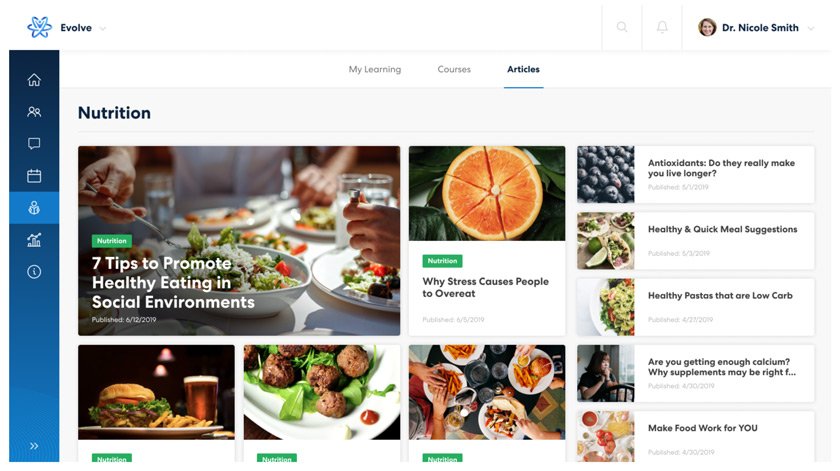The image depicts a website page dedicated to food and nutrition. The top-left corner displays a logo featuring a blue star-shaped figure with a smiley face, alongside the site's name "Evolve". On the top right, there is a picture of Dr. Nicole Smith. 

Beneath this, three main headings are arranged: "My Learning", "Courses", and "Articles", with “Articles” currently selected, highlighted, and bolded for emphasis. Running along the left-hand side against a blue sidebar are several icons representing various functions: a house (home), a people icon, a chat box, a calendar, and more.

Central to the screen are numerous panels, each depicting different meal presentations, accompanied by green buttons labeled 'nutrition.' These panels feature headings such as "Seven Tips to Promote Healthy Eating and Social Environments" and "Why Stress Causes People to Overeat".

To the right, additional article titles are listed, including "Healthy and Quick Meal Suggestions," "Healthy Pastas that are Low Carb," and "Make Food Work for You". The layout is clean, organized, and visually appealing, focusing on providing users with informative and practical content on healthy eating and nutrition.